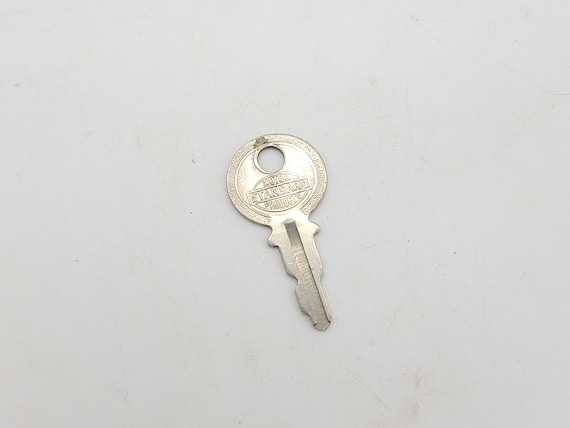This image features a small silver key centrally placed on a light gray surface that appears to be a tabletop. The key itself is oriented diagonally, with the top leaning slightly to the left and the bottom to the right. The tabletop surface has visible signs of wear, including brown scratch marks and slight discolorations. The key is metallic and light gray in color, with a round head that has a circular hole punched out at the top, suitable for attaching to a keychain. Below the hole, there is engraved text, including a rectangular box in the middle with the word "STANDARD" and some additional, albeit unreadable, text likely indicating numbers both above the rectangle and curving along the bottom edge of the circular head. The bottom part of the key features a vertical, jagged-edged blade designed for locking mechanisms.